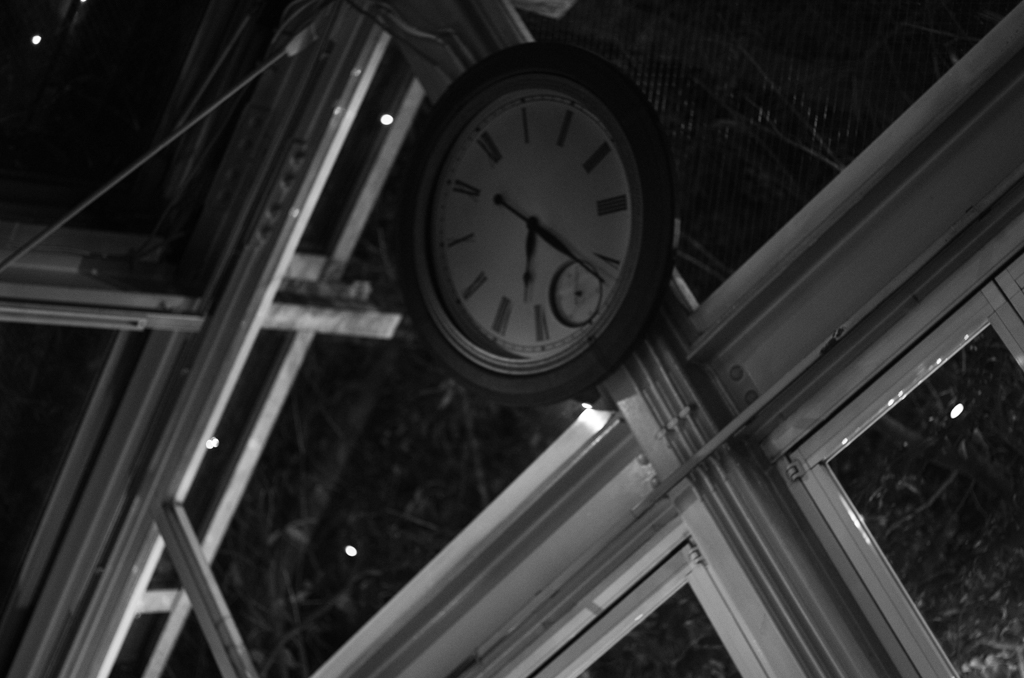In this black and white photograph, we observe an interior space characterized by extensive use of glass panels providing a view of an exterior adorned with what appears to be branches or leaves of trees. Dominating the image is a large, classic wall clock mounted high towards where the ceiling meets the wall. The clock, encased in a black circular trim, features Roman numerals and a smaller dial at the position where the six would typically be, resembling a chronograph. The clock’s hands, including the hour, minute, and second hand, are all black in color, contrasting sharply against the white background of the clock face. The structure features prominent white trim and borders, particularly around glass-panelled doors below the clock, allowing for transparency and visibility to the outside. The ceiling appears dark and somewhat transparent, adding to the open, airy ambiance of the space. This could be an interior shot of a building with a large glass facade, perhaps reminiscent of a greenhouse or a modern fire station with roll-up metal windows and doors. The overall view is slightly tilted, suggesting a dynamic perspective that emphasizes the height and structure within this unique architectural setting.